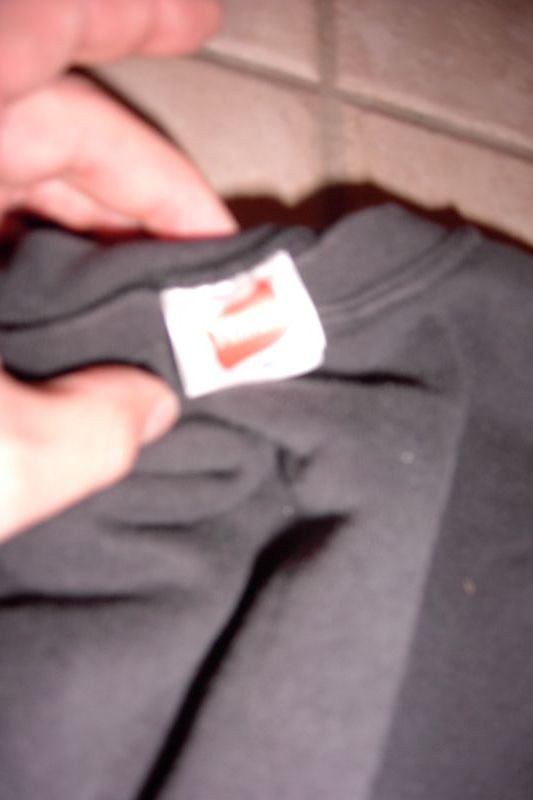In the photograph, a person's hand is visible resting on a black article of clothing. The image has an oversaturated appearance due to a bright camera flash reflecting off the fabric. The garment is laid on a tan tiled floor, with darker grout lines visible at the top. The shadow of the shirt is cast on the floor, adding depth to the scene. A white tag with a red section and white text is sewn into the collar. The stitching along the collar is noticeable. The black fabric of the clothing is speckled with visible lint and dirt, including a white-colored piece and another that is a very pale orange hue.